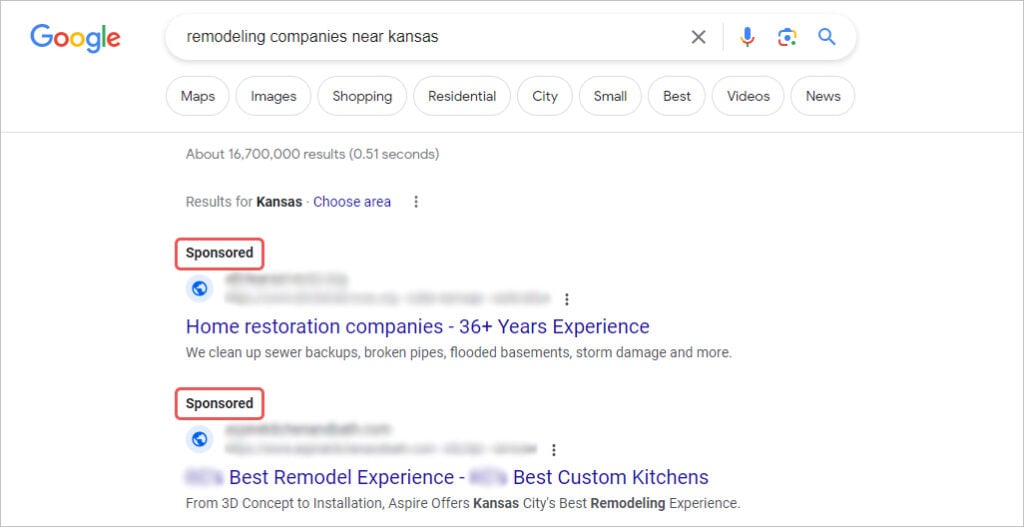This is a detailed and cleaned-up caption for the provided image:

The image is a screenshot of a Google search results page presented in a rectangular format. In the upper left corner, the iconic Google logo is displayed, consisting of the letters "G-o-o-g-l-e" in vibrant colors: blue for 'G', red for 'o', yellow for the second 'o', blue for 'g', green for 'l', and red for 'e'. Centrally located on the page is the signature Google search bar, rectangular with rounded edges, containing the query "remodeling companies near Kansas" typed in black text.

Below the search bar, there are several smaller rectangular buttons outlined in gray. These buttons, each containing central black text, provide additional search options labeled as: Maps, Images, Shopping, Residential, City, Small, Best, Videos, and News.

Further down the page, the search results are displayed. A gray text indicates that there are approximately 16,700,000 results found in 0.51 seconds. The top of the search results includes a couple of titles within red rectangular outlines, identifying them as sponsored links. The bolded black text within the red outlines reads "Sponsored" to differentiate these from the organic search results.